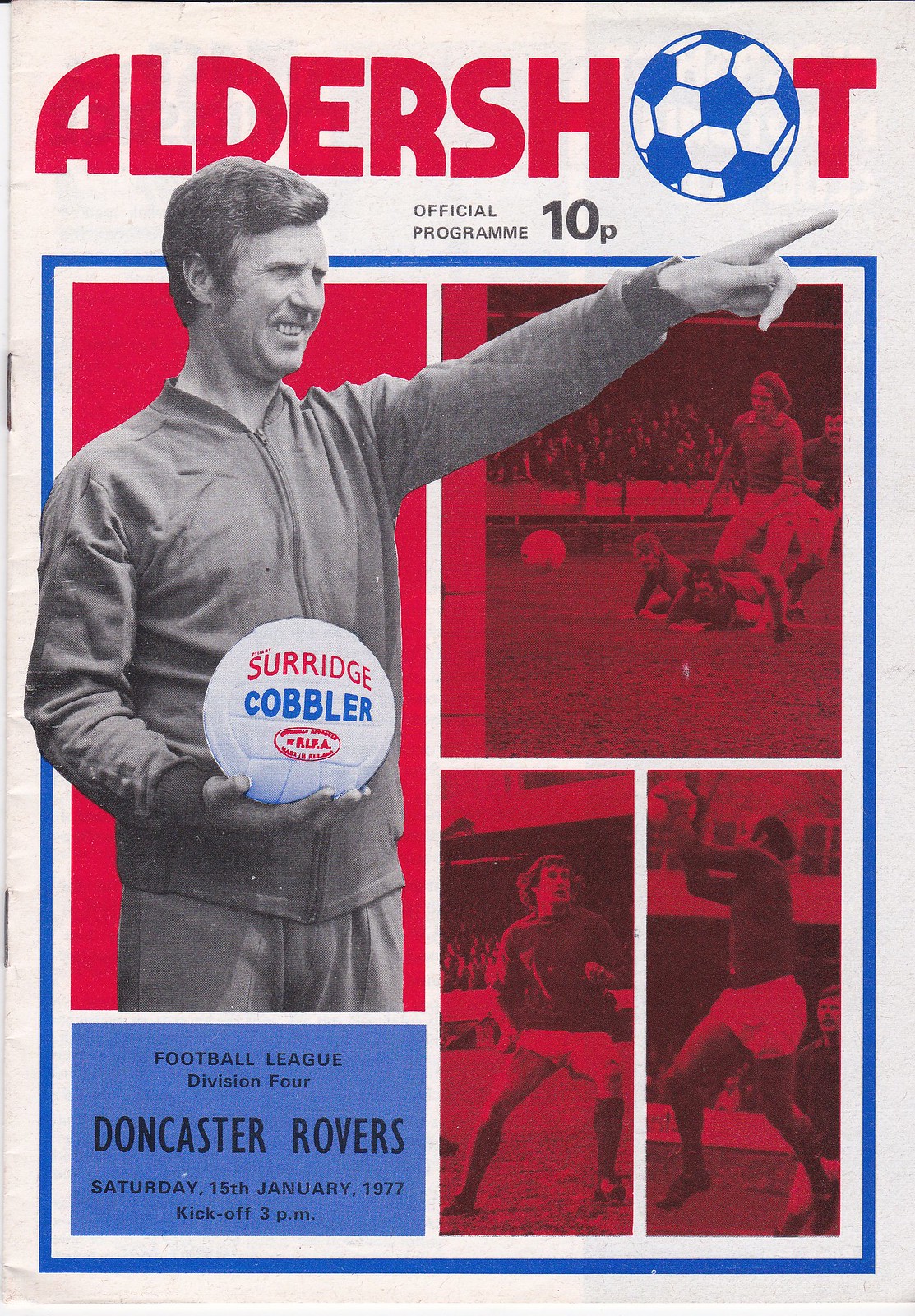This is a scan of a vintage magazine cover titled "Aldershot," with the 'O' stylized as a blue and white soccer ball. The cover reads "Official Program 10-P" and prominently features a black-and-white image of a man pointing while holding a soccer ball labeled "Surridge Cobbler." To the right, there are several monochromatic photographs in shades of red and dark red, depicting players engaged in a soccer match. The bottom of the cover, framed by a blue border, announces "Football League Division IV, Doncaster Rovers, Saturday, 15th January 1977, kickoff at 3pm." The magazine has staples visible along the left edge, indicating it's a thin, staple-bound program. The background is predominantly white, enhancing the retro aesthetic of this 1977 soccer program.